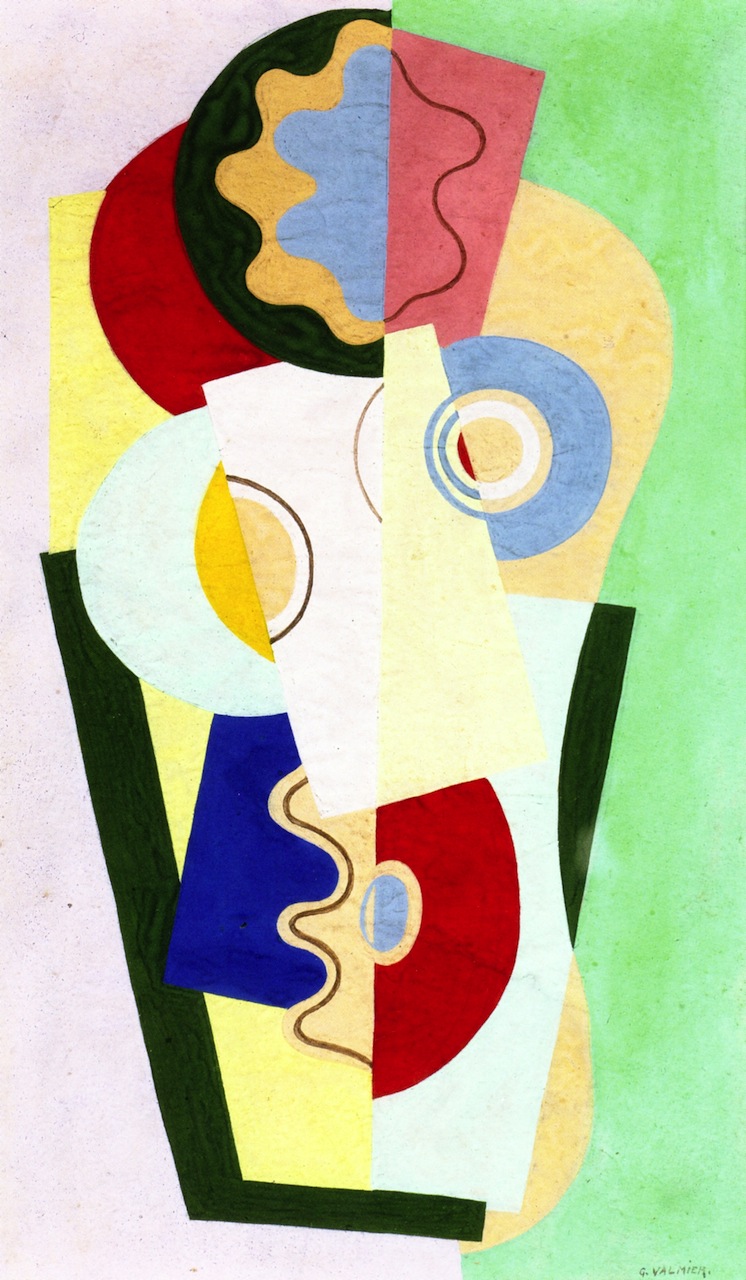The artwork is an abstract painting with a style reminiscent of Picasso, featuring a mix of blocks and circular forms in an array of vibrant colors. The rectangular canvas, taller than it is wide, is split down the center. The left half boasts a light pink background, while the right half features a green background that darkens from bottom to top, providing a watercolor-like texture. 

In the lower left quadrant, a dark green shape resembling an L anchors the composition. Within the left part of this L, a tan block contains a blue, rounded, capital E-like figure. Adjacent to this is a white block with a red half-circle and a light blue oval. Above these elements, a horizontally placed white and light yellow rectangle hosts an egg yolk-like shape on its left side and a light blue half-circle overlapping a white half-circle on its right. 

Up above, on the right side of the center line, a red rectangle with a black squiggly line contrasts with a black half-circle to its left, which contains blue and yellow blotches. Just below this, a red half-circle nestles in the lower right corner. The artist has signed the piece with "G. Valmier" in the bottom left.

Overall, the composition is punctuated with half-circles, concentric shapes, and squiggly lines, blending fluidly into the divided color scheme.